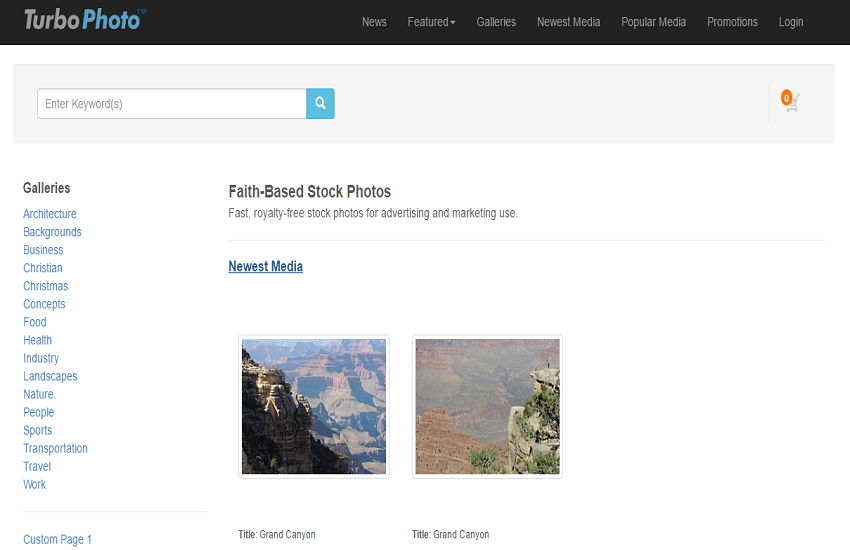The image showcases the homepage of TurboPhoto, a website specializing in stock images. At the top of the page, an extensive horizontal menu bar is prominently featured. On the far left of this bar, the site’s name, "TurboPhoto," is displayed. To its right, the menu options are listed sequentially: News, Featured, Galleries, Newest Media, Popular Media, Promotions, and Login.

Beneath the menu bar sits a search bar that allows users to input keywords to find specific stock images. On the left side of the page, there is a vertical list of stock photo categories, including Architecture, Backgrounds, Business, Christian, Christmas, Concepts, Food, Health, Industry, Landscapes, Nature, People, Sports, Transportation, Travel, and Work.

Towards the bottom, the site mentions "Custom Page 1." The main content displayed focuses on faith-based stock photos, emphasizing the availability of fast, royalty-free stock images suitable for advertising and marketing. It also highlights the "Newest Media" section, which features two stock images of the Grand Canyon. Both images capture the majestic beauty of this iconic landmark.

Overall, the layout and organization of the TurboPhoto website are designed to offer users easy navigation and access to a wide variety of stock photos for various purposes.